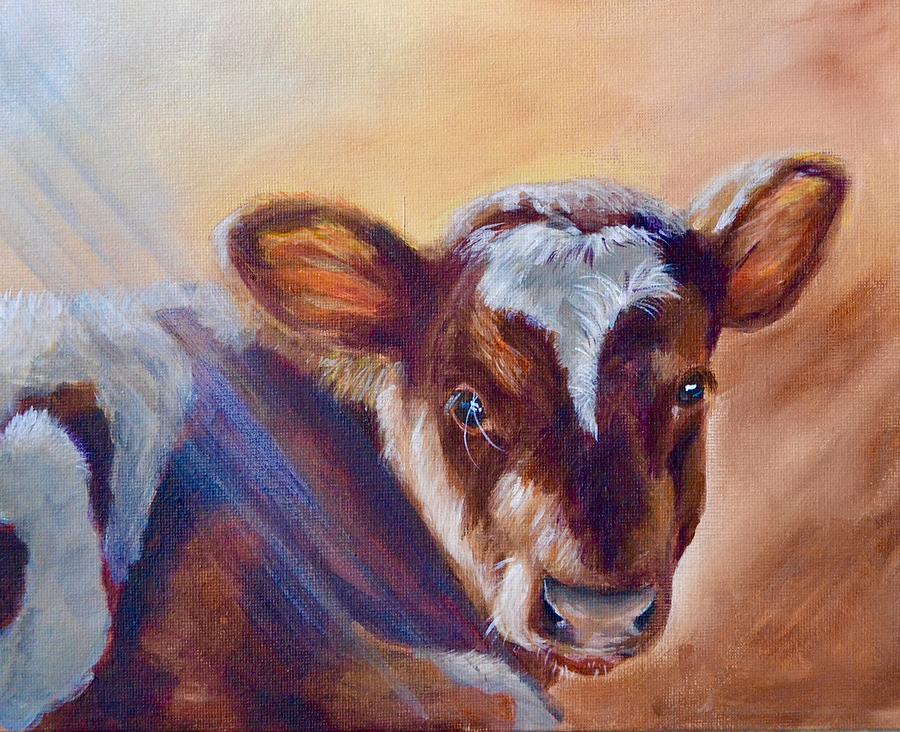This image showcases a unique and detailed watercolor painting of a baby cow, or calf, characterized by its endearing and innocent appearance. The calf's fur is a blend of brown, white, and black, with noticeable patches including a prominent white streak extending from its forehead down between its expressive, shiny black eyes. The nose features a striking combination of black, white, and orange hues, appearing larger than expected. The calf's ears are predominantly brown, accentuated with touches of beige and red, while one eye is highlighted with white eyelashes. The painting captures the calf from the head to just part of the shoulder, emphasizing its youthful features. It gazes directly at the viewer with a neutral, almost contemplative expression. The background is a warm mix of muted colors, including pale blue, white, vanilla, and varying shades of orange and brown, with a touch of purple or blue swirl subtly intertwined. The canvas lacks any text or signature, allowing the intricate details and harmonious color palette to speak for themselves.